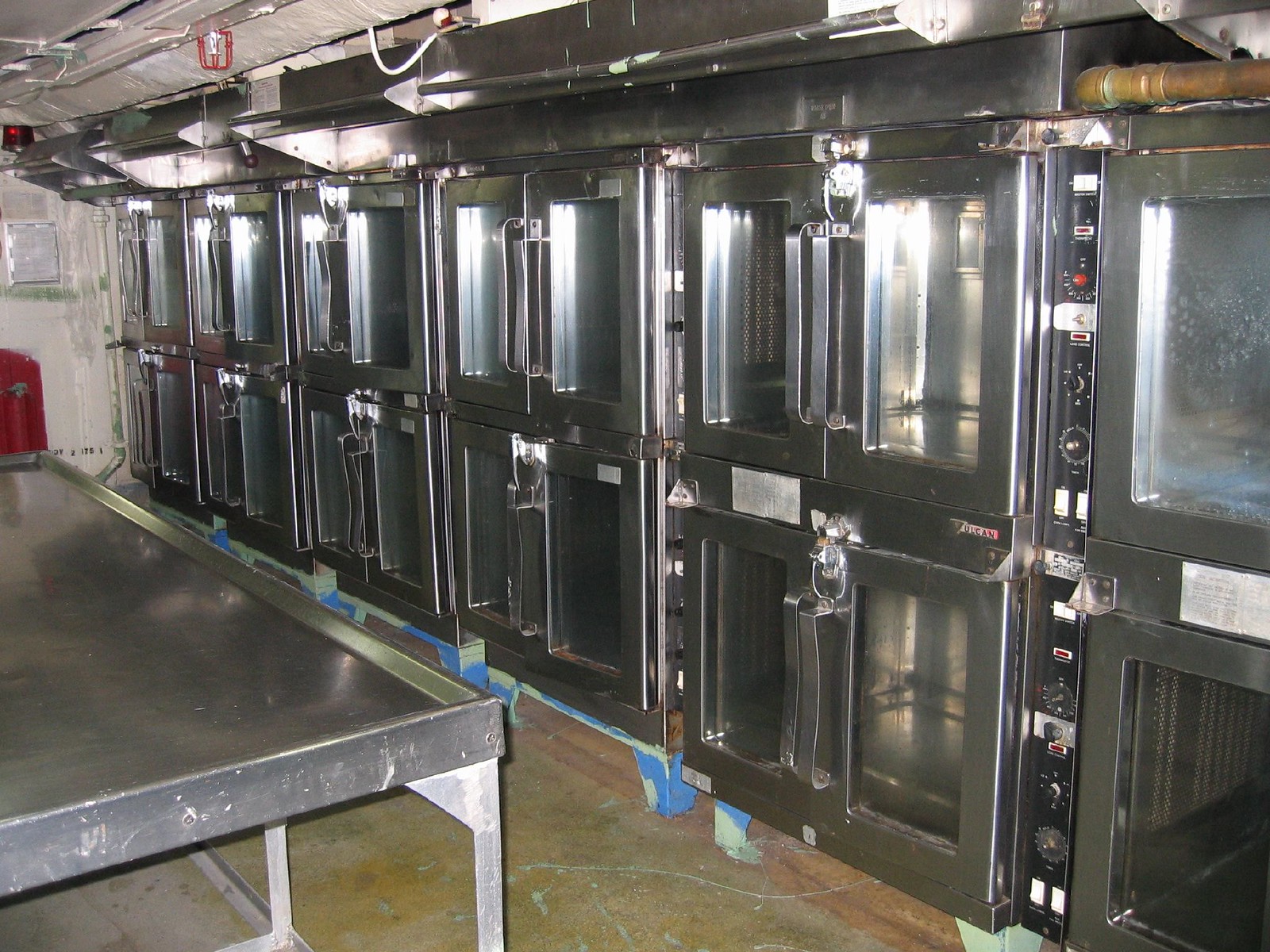This color photograph captures the detailed interior of what appears to be an industrial kitchen, possibly a bakery or a laboratory. The main focus is a bank of large, stainless steel ovens, tightly aligned against a white back wall and topping out in two rows of five ovens each, for a total of ten visible units. Each oven is equipped with clear glass viewing panes, black control panels, and vertical stainless steel handles opening from the center. The ovens seem to be inactive, with pristine, empty interiors.

Above, the ceiling is a metallic silver color, featuring a clearly visible fire suppressant system with sprinkler heads and pipes running along it. The floor is a well-worn, beige concrete with visible cracks and scratches, adding an aged appearance to the room.

To the right of the image is a spacious, chrome metal work table. This table is about waist-high, with a shiny, reflective surface and a raised ridge around its edges, providing a practical workspace that remains uncluttered. Blue tape or paint is noticeable on some of the oven legs, hinting at marks for repositioning or alignment.

Overall, the detailed and well-arranged layout suggests an industrial environment, equipped and ready for high-volume food preparation or culinary experiments.